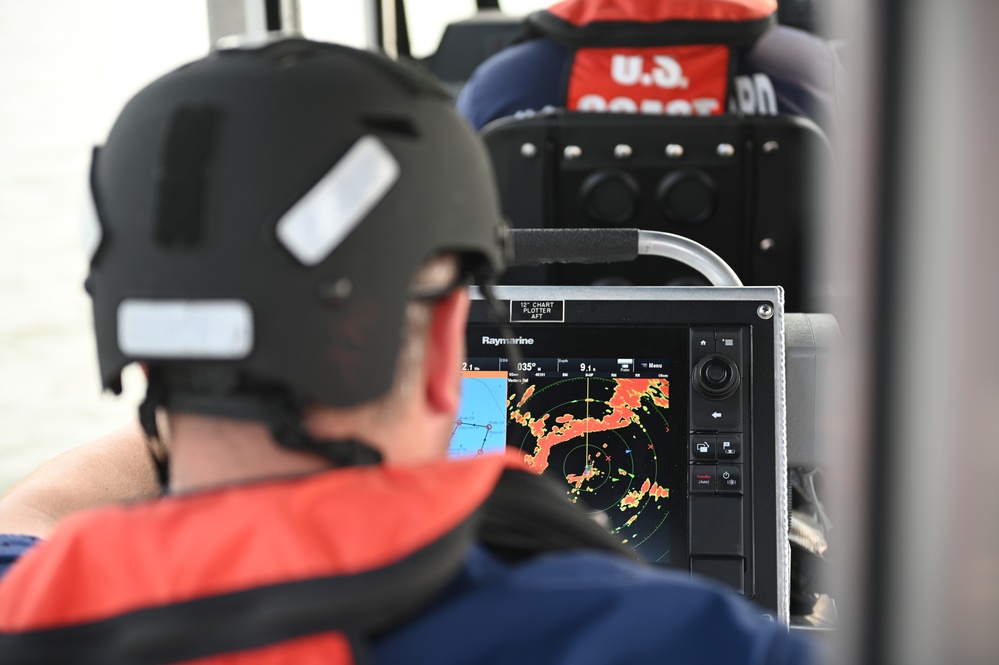This photograph captures a man engaged in what appears to be a monitoring task. The man is seated and viewed from behind, wearing a black helmet and a blue jacket with an orange collar. In front of him is a monitor displaying what looks like a radar screen, featuring black as the background with yellow rings and irregular shapes resembling clouds, possibly indicating weather patterns. He appears focused on the screen, perhaps interpreting the radar data. There's another man seated directly in front of him, partially visible, adorned in a red vest that reads "U.S. Coast Guard," suggesting a similar role or environment, likely within a maritime or operational setting. The setting hints at a boat or similar vehicle, accentuating the functional nature of their activities.